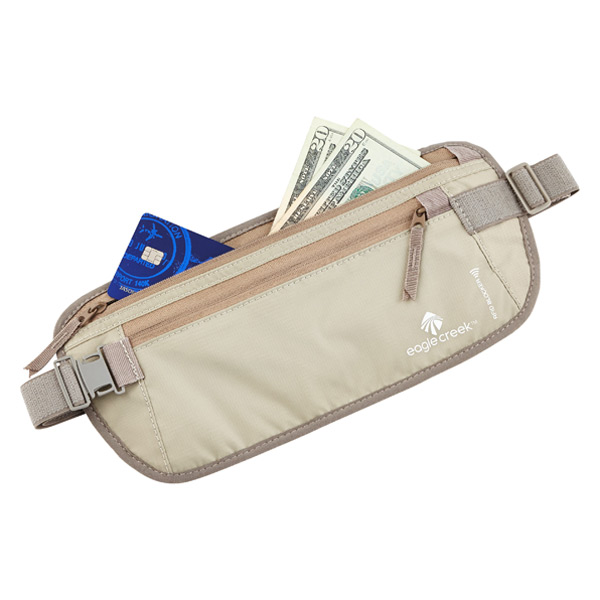This is an image of a khaki-colored fanny pack by Eagle Creek, prominently displayed against a white background, suggesting it is likely an advertisement for the brand. The fanny pack has a front zipper in a darker beige shade, and on the bottom right corner, it features the Eagle Creek logo and name in white, along with a diamond-shaped logo with lines.

The main pocket is open, revealing a blue credit card diagonally protruding from the left side. The credit card is detailed with a silver chip and an airplane icon, along with the name "Jason" visible. On the right side of the main pocket, two U.S. $20 bills are similarly sticking out. Additionally, there is mention of RFID-blocking capabilities, suggesting the pouch provides protection against wireless theft.

The fanny pack has gray straps with a clasp on the left-hand side and a buckle on the right-hand side. There is also a secondary zipper located to the left of the blue credit card. This detailed arrangement emphasizes the practical uses of the fanny pack, showcasing its capacity to securely hold and organize personal items like money and credit cards.